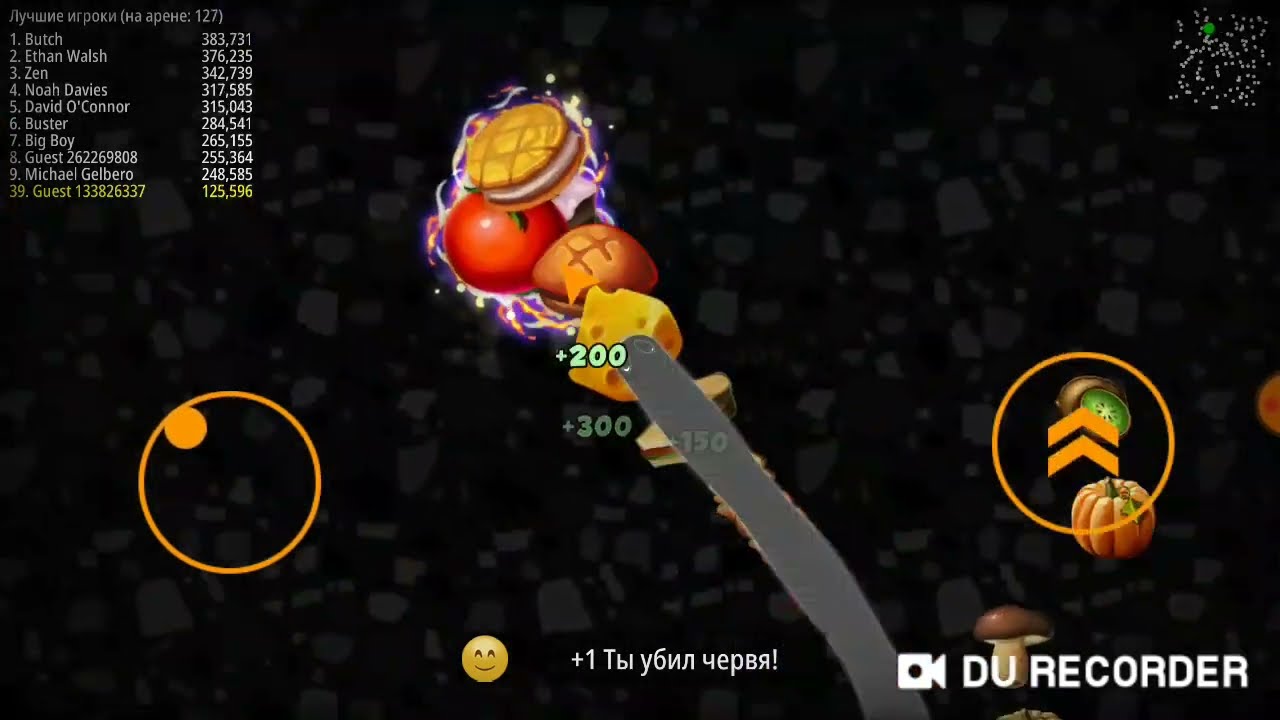The screenshot depicts a video game interface against a dark background speckled with white or gray stones. Dominating the center is a gray line, along which various food items are positioned: starting from the end of the line, there is a chunk of cheese, followed by a piece of bread, a red tomato, and finally, a yellow cookie with a white cream center. Numbers such as "+200," "+300," and "150" are displayed near these items.

In the upper left corner, a leaderboard lists player names, including Butch, Ethan Walsh, Zen, Noah Davies, David O'Connor, Buster, Big Boy, Guest 262269808, Michael Gerbo, and Guest 133826337, with corresponding scores arranged from highest to lowest. At the bottom corners of the screen, two orange circles represent control buttons: the left circle, containing a smaller orange circle inside, probably for movement controls, and the right circle with two upward-pointing wedges, likely the attack or slash control.

At the center bottom, white text displays "+1 TBI" followed by characters in Russian, beginning with "Y" and the number "6," ending with an exclamation mark. Additionally, an emoji of a smiley face with its eyes closed is situated alongside a camera icon labeled "DU RECORDER" in white, uppercase letters at the bottom right corner.